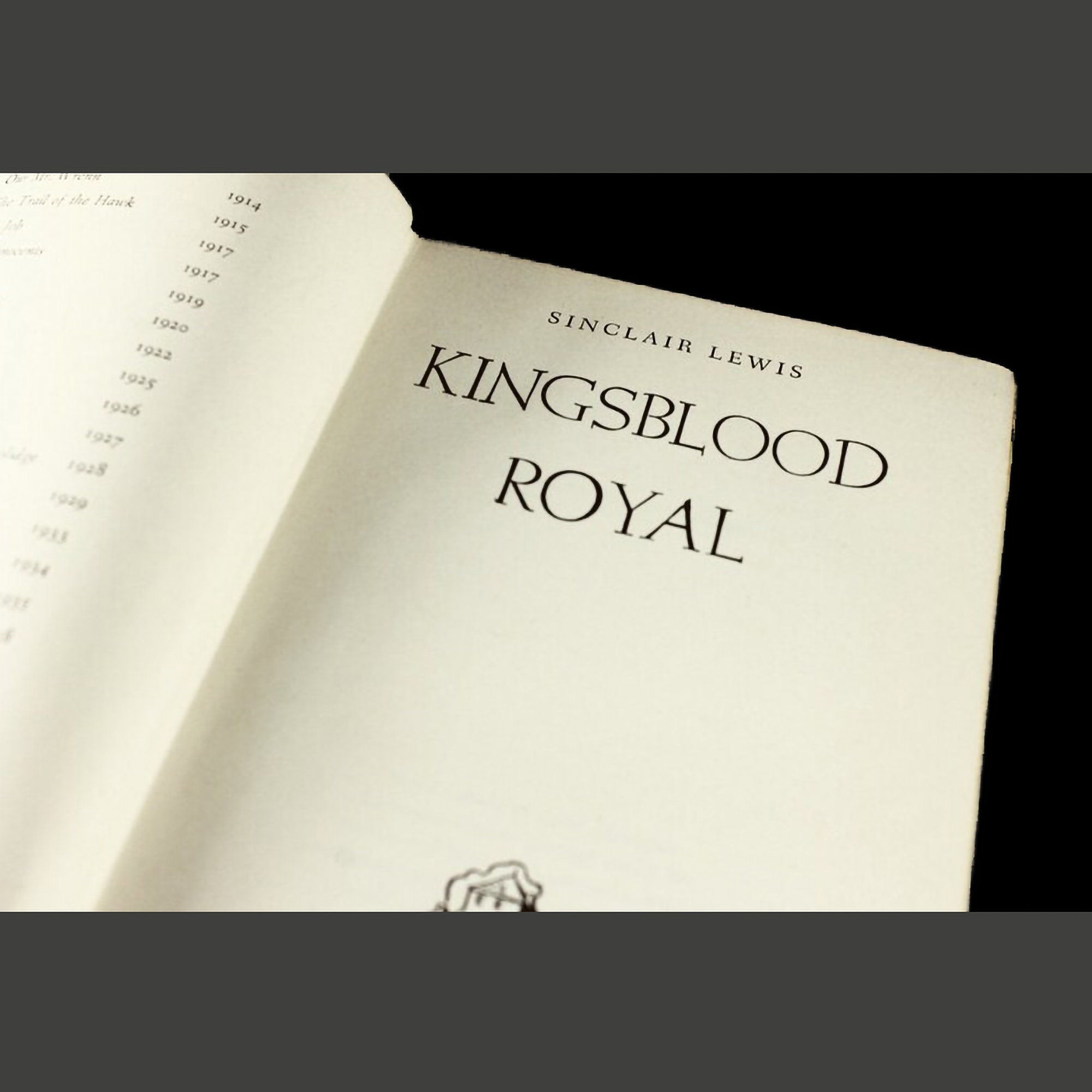The image features an open book set against a black background. The book is slightly angled downward, revealing the title page on the right side. The title page, printed in black text on creamy white paper, prominently displays "KING'S BLOOD ROYAL" in large capital letters. Above the title, in smaller print, is the author's name, Sinclair Lewis. At the bottom of the title page, there is a small emblem resembling a house, suggesting it might be published by Random House. On the left-hand side, partially visible, is the preceding page featuring a list of years, likely corresponding to other works by the author, including 1914, 1915, 1917, 1919, 1920, 1922, and 1934. The book's positioning leaves its binding and covers unseen, making it unclear whether it is hardbound or softbound.